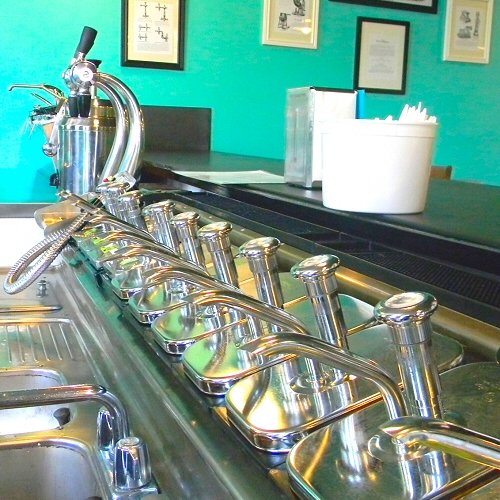The vibrant interior of the establishment, which could be a bar, an ice cream parlor, or a soda fountain, exudes a charming retro vibe. Dominating the foreground are shiny, silver condiment containers, intricately aligned from the bottom right towards the middle left, their polished surfaces gleaming under the light. Each container, around nine or ten in total, features a push-down knob and spout for easy dispensing. Adjacent to the containers, a sleek black counter runs diagonally with a white tub holding utensils and napkins neatly placed on it. A contrasting turquoise wall forms the backdrop, adorned with framed pictures and certificates, adding an eclectic touch. Positioned towards the bottom left of the image are a few faucet handles, hinting at sink areas integral to the setup. The countertop also extends into the background, housing additional containers that complement the overall organized chaos of the scene. The palette of colors throughout the image includes teal, mint green, silver, black, white, blue, brown, beige, and tan, creating a visually stimulating and inviting atmosphere.